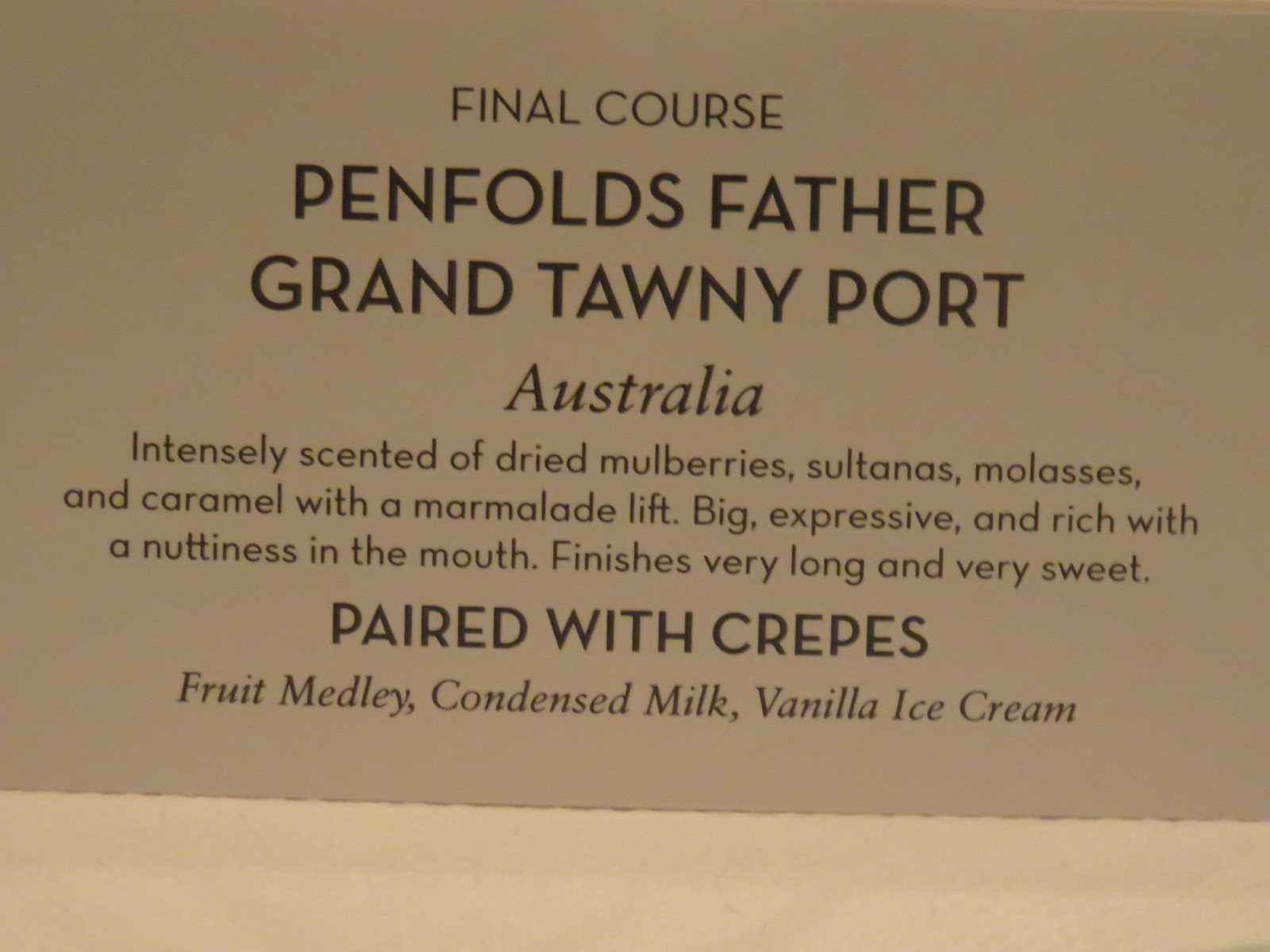The image depicts a sandy-colored card positioned on a wooden table, with dark brown text that reads at the top, "FINAL COURSE" in black capital letters. Below that, in larger capital letters, it says, "PENFOLDS FATHER GRAND TAWNY PORT." Underneath, it states "Australia," followed by detailed sensory notes: "Intensely scented of dried mulberries, sultanas, molasses, and caramel, with a marmalade lift. Big, expressive, and rich, with a nuttiness in the mouth. Finishes very long and very sweet." The card also mentions pairings: "Paired with crepes, fruit medley, condensed milk, and vanilla ice cream." The text varies between capitalized and regular fonts, offering a comprehensive description likely for a wine tasting or final course dessert pairing.